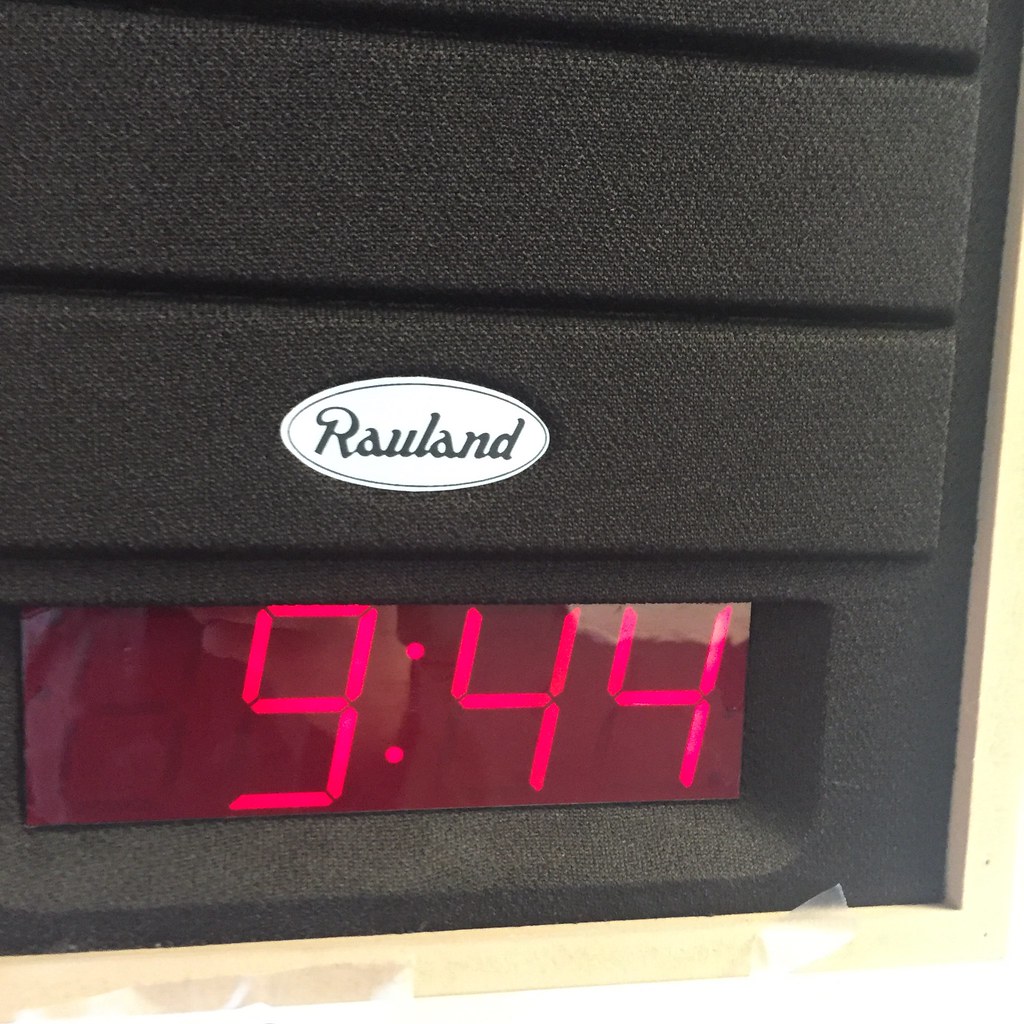The photograph depicts a black electronic device, which appears to be part of an entertainment system or a speaker. The device features a textured, fabric-covered surface with horizontal sections. The top half showcases three large rectangular sections with grooves, and on the middle section, there is an oval white background with the name "Rauland" written in stylized black text. Below this section, a large rectangular digital clock display shows the time "9:44" in bright red numbers against a reddish background. This display is also slightly reflective, revealing a faint reflection of the person taking the photograph. The device is mounted on a light brown, wood-like shelf structure, which is partially visible, indicating that it might be part of a larger setup.